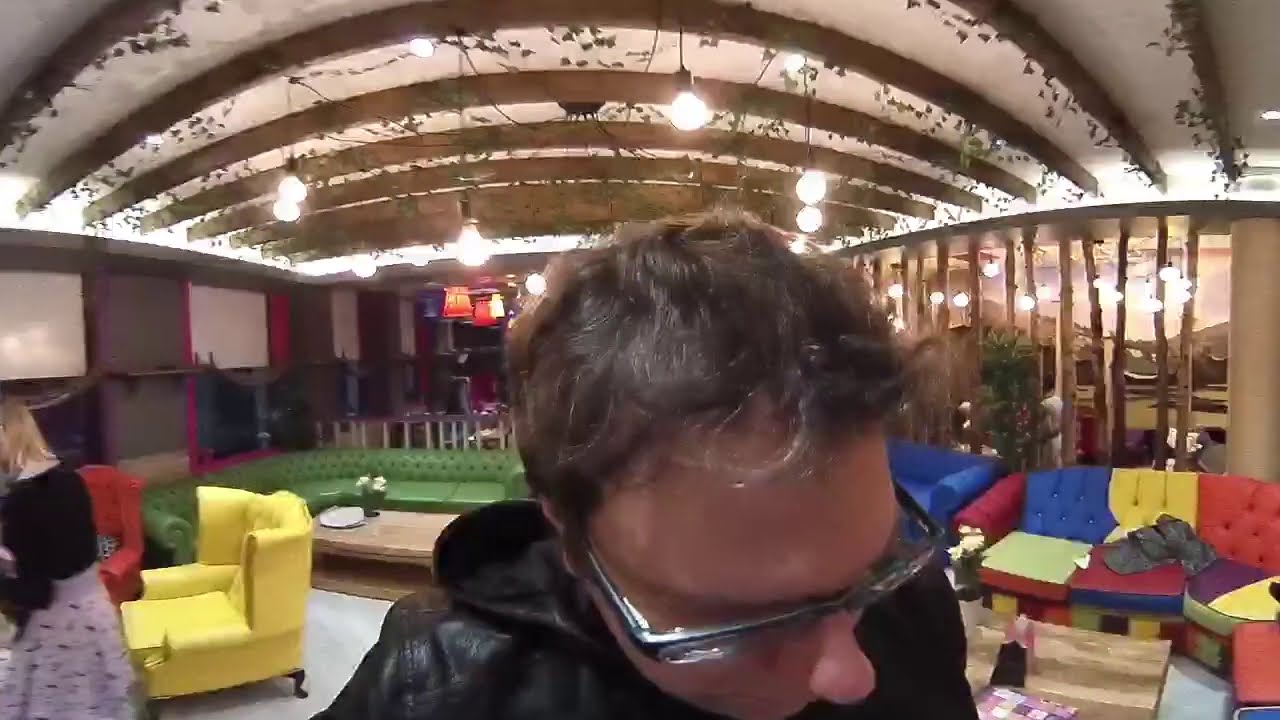In the foreground of the image, there is a close-up of a middle-aged man with short brown hair wearing glasses and a black leather jacket. He is looking down and to the right. Behind him, inside a well-lit lounge area, the ceiling is vaulted with white panels and decorated with hanging light bulbs suspended from wires. The ceiling also features brown wooden panels and some leaf decorations. The seating arrangements in the room include a large L-shaped green sofa around a wooden table, located to the man's left. Additionally, there is a red and yellow chair near the bottom left corner where a woman is standing. She has blonde hair, is wearing a black top and a pink dotted skirt, but her face is not visible. The lounge area is filled with brightly colored furniture, including yellow, red, blue, and green sofas, along with some tables that have flower arrangements and plates on them. There are many windows along the right side of the image, which is also lined with more colorful seating, contributing to the vibrant ambiance of the room.